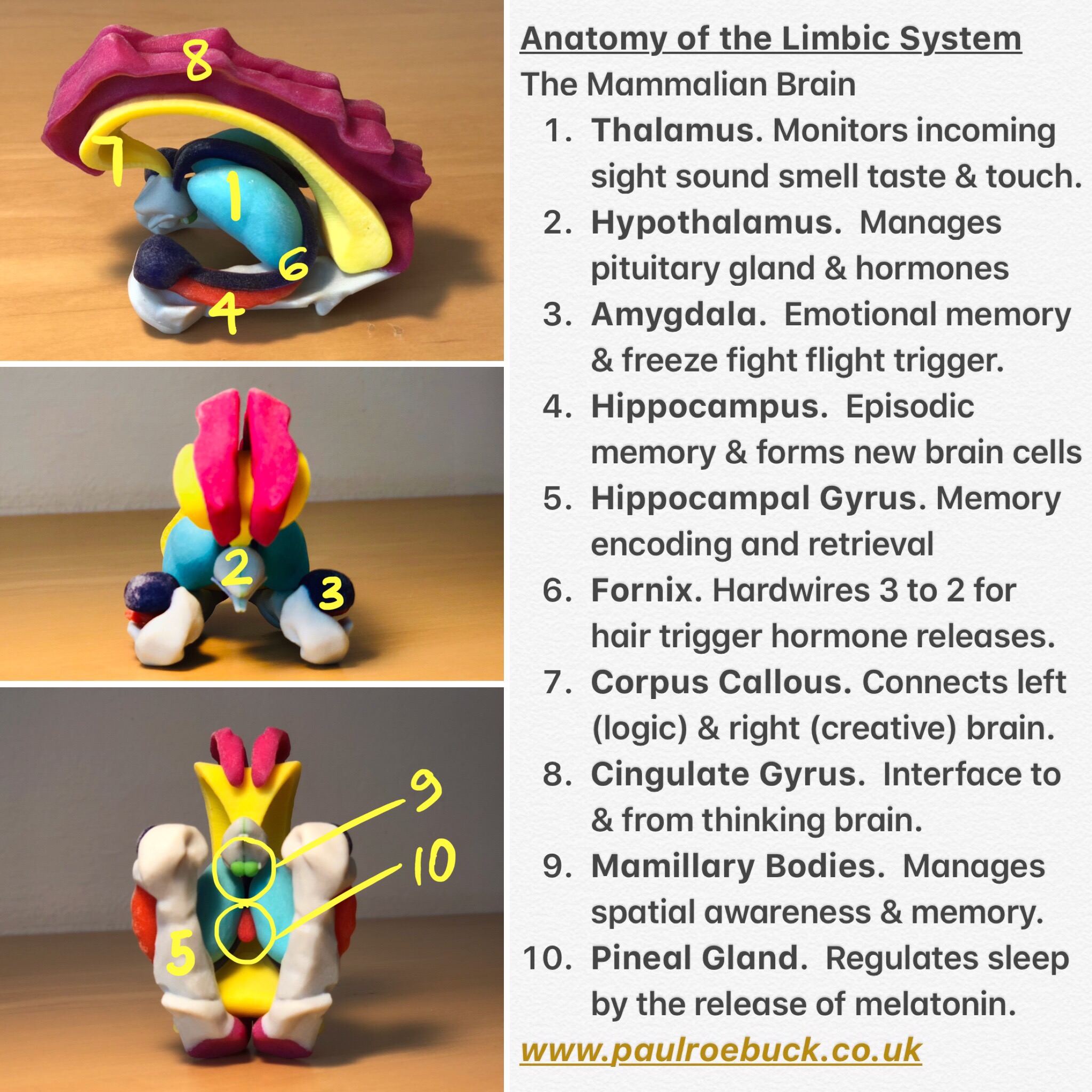The image is a large, borderless square divided into two distinct sections. On the left side, there are three vertically stacked rectangles displayed against a brown counter or table with an off-white wall in the background. Each rectangle contains colorful, clay-like models representing different parts of the limbic system. The top rectangle showcases a model predominated by purple and yellow colors, featuring an open mouth with objects inside and hand-drawn yellow numbers. The middle rectangle presents a similar model but displayed from a different angle or position. The bottom rectangle also contains this model, reconfigured into another form.

On the right side of the image, there is a long vertical rectangle with a light gray background. This section contains a detailed textual description titled "Anatomy of the Limbic System" followed by "The Mammalian Brain." It lists and describes ten parts of the limbic system in vertical alignment, each accompanied by a short sentence. The parts are: 1) Thalamus, 2) Hypothalamus, 3) Amygdala, 4) Hippocampus, 5) Hippocampal Gyrus, 6) Fornix, 7) Corpus Callosum, 8) Cingulate Gyrus, 9) Mammillary Bodies, and 10) Pineal Gland. The bottom of this list mentions a website where viewers can learn more about the limbic system.

Together, these elements create a detailed visual and textual guide to the anatomy of the limbic system using colorful, possibly 3D-printed or clay models to illustrate the parts and their arrangement within the brain.